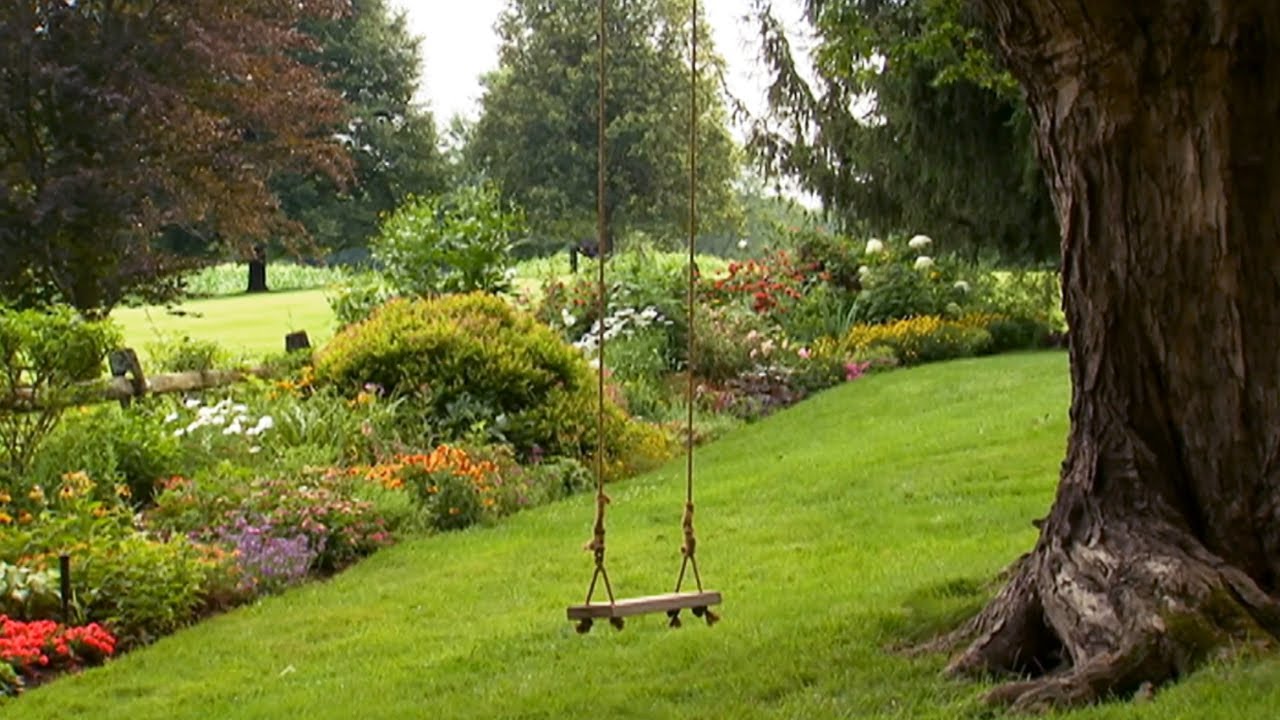The image captures a picturesque backyard or park-like setting dominated by a majestic, thick-trunked tree. Hanging from the tree's sturdy branches is a wooden swing, suspended by ropes on either side, and featuring a light beige color. The lush, vibrant green lawn beneath and around the swing is impeccably maintained, creating a neat and inviting atmosphere.

In front of the tree, a beautifully cultivated flower garden bursts with a kaleidoscope of colors. The garden features an array of flowers including reds, whites, yellows, pinks, purples, oranges, and light lavenders, intermingled among various bushes and plants. This lively mix of blossoms adds a touch of elegance and vibrancy to the serene setting.

Behind this colorful spectacle stands a rustic wooden log fence, with additional lawn and larger trees visible beyond it. The overall composition places the swing at the heart of the image, inviting one to enjoy the peaceful charm of this flower-filled, green oasis surrounded by nature's beauty.